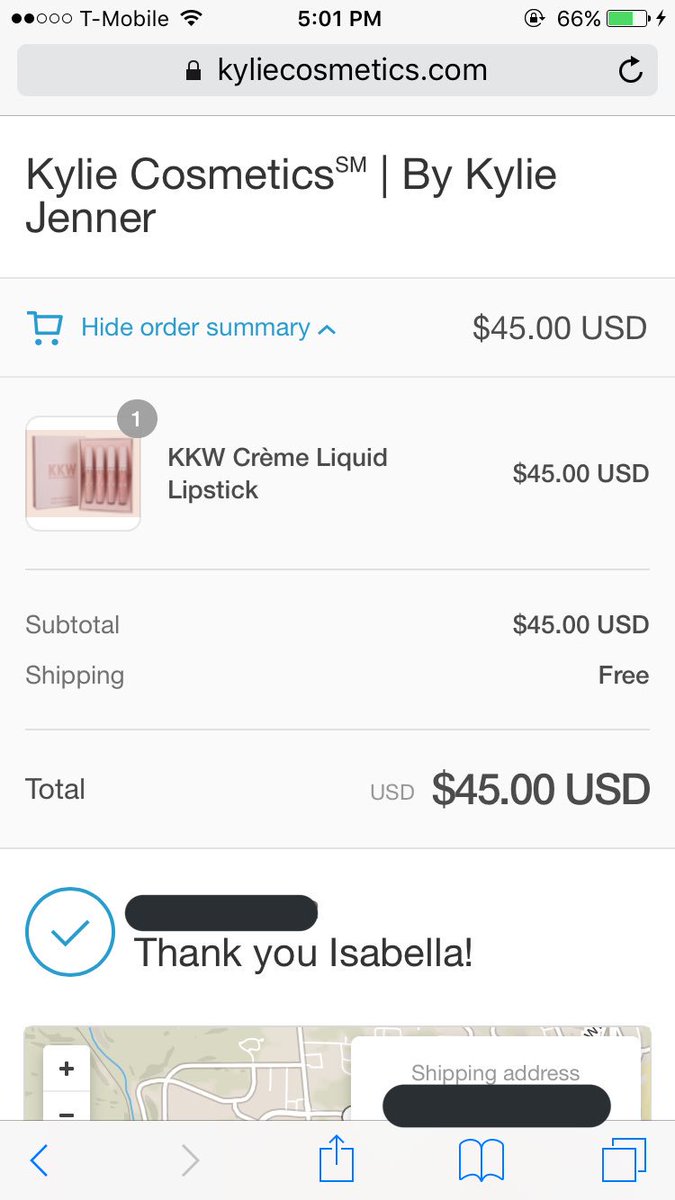The image depicts a mobile phone screen displaying the Kylie Cosmetics website, known for its beauty products. The device is connected to the T-Mobile network, with the battery level at 66% and the time indicated as 5:01 p.m. The URL visible on the screen is KylieCosmetics.com. Prominently displayed on the website are the words "Kylie Cosmetics Jenner" in large black letters, followed by the phrase "SM by Kylie."

A cart summary shows an order totaling $45 USD for the KKW Cream Liquid Lipstick set, which includes four lipsticks packaged in a pink box. The product image is clearly visible, displaying part of Kylie Jenner's name. The subtotal of the order is listed as $45 USD, with free shipping prominently noted, making the total cost exactly $45 USD.

Certain personal information, including the shipping address and potentially sensitive details, have been blacked out. A white circle with a blue outline and a blue check mark accompanies a message reading "Thank you Isabella!" followed by an exclamation point, indicating appreciation for the customer's purchase. A map is also partially visible, further indicating the shipping details that have been obscured for privacy.